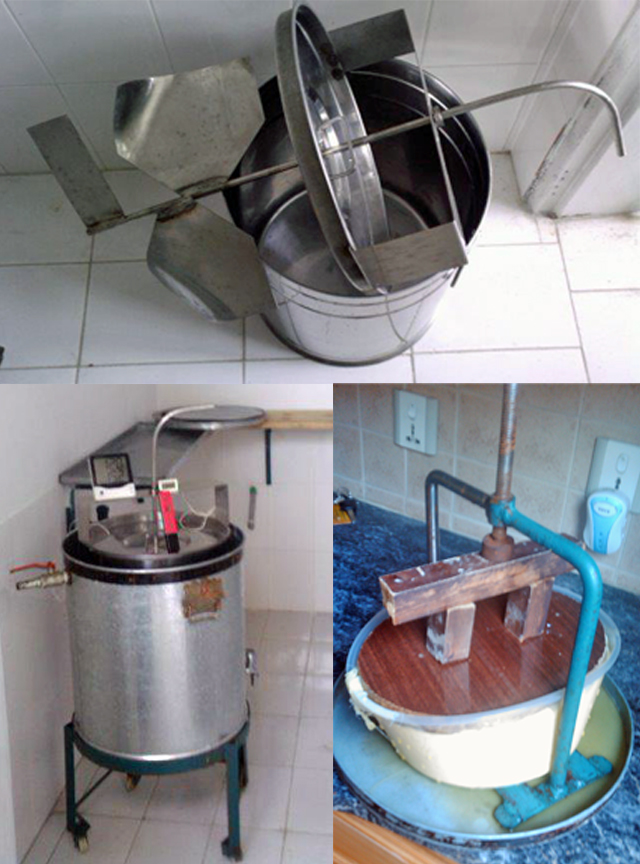The image is composed of three vertically aligned rectangular sub-images. The top image depicts the interior of a metal tin or bucket with a rod lying across it, featuring a lid in the middle and blades at the end. This setup lies on a white tiled floor with a white tiled wall behind it, adjacent to a doorway. The lower left image shows a cylindrical metal tin on black legs with wheels. This tin has a black border around its top, a possible thermometer inside, and a small digital screen. The lid of this tin is positioned on a wooden shelf attached to a white tiled wall. The lower right image reveals a blue granite countertop with a metal tray on which a white bucket sits. Atop the bucket is a circular wood piece, and a metal gadget with an upward rod and a blue bar descends on its side. The overall scene incorporates colors like metallic gray, walnut, blue, light blue, white, black, and red. The objects appear to be various kitchen utensils or appliances, suggesting a kitchen environment.